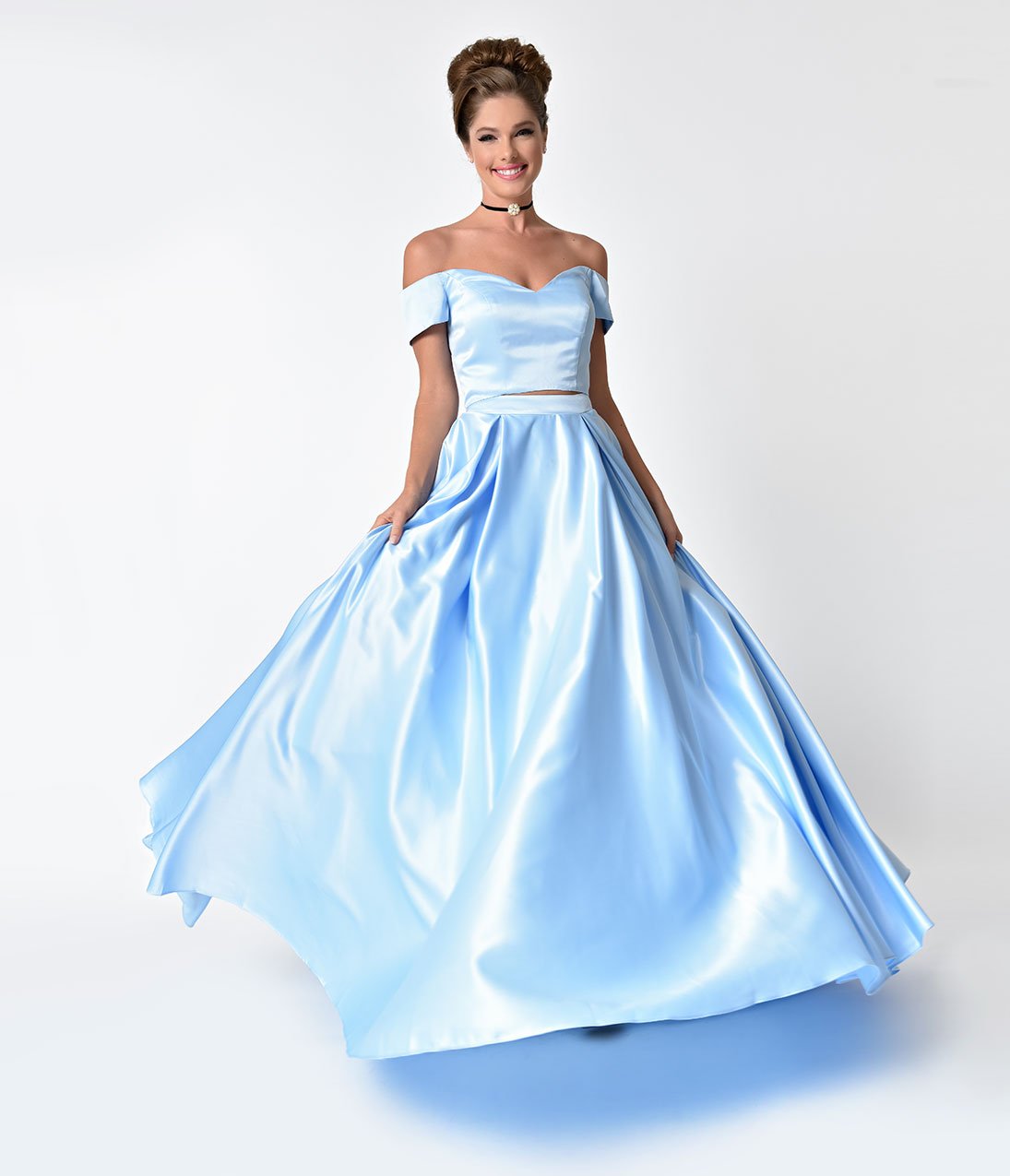In this image, a young brunette female model is posing gracefully in a princess-like Cinderella gown. Her hair is styled elegantly in large, voluminous curled buns atop her head, adding to her majestic appearance. She has a natural, radiant smile enhanced by subtle makeup. Around her neck, she wears a simple black choker adorned with a white or silver diamond, providing a touch of classic elegance.

Her gown is a light, baby blue color, reminiscent of Cinderella's iconic ball gown. The off-shoulder satin material glistens under the light, showcasing the tube top that seamlessly transitions into a full, flowy skirt. The skirt is puffed up to create a dramatic, voluminous effect, and the entire gown possesses a shiny, satin-like quality. The model stands against a clean, white background, with her hands gently holding the skirt, adding a whimsical, fairy-tale touch to the scene. This enchanting setup makes her look like a true princess.